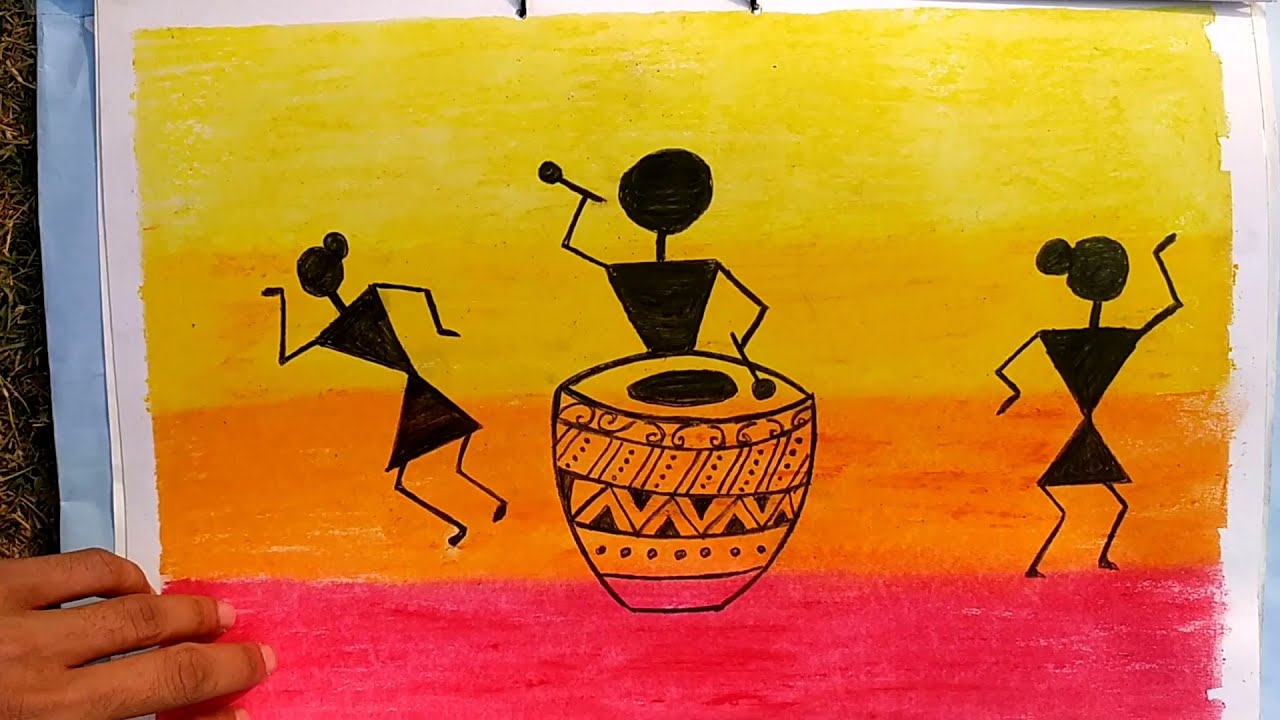In this image, we see a vibrant, abstract painting that appears to depict an African-inspired scene. The background features four distinct horizontal bands of color transitioning from pink at the bottom, to orange in the middle, and to yellow at the top. Superimposed on this colorful backdrop are black silhouettes that resemble stick figures with more defined triangle-shaped bodies. The central figure is a man playing a stylized African drum detailed with various patterns including stripes, dots, triangles, and curly designs at the top. His body is designed with an upside-down triangle for the torso and spherical shapes for the head and hands. On either side of the drummer, there are two women figures who appear to be dancing; their bodies also consist of triangles with stick arms and legs, and they have small black circles at the back of their heads, suggesting tied-back hair. In the bottom left corner of the image, three fingers are visible, holding the painting, indicating that this is a photograph of the artwork rather than the artwork itself. The painting uses no text and combines elements like colored pencil or crayon for the vivid background and pen for the detailed black silhouettes. The overall composition gives a dynamic and lively impression, celebrating movement and cultural motifs.